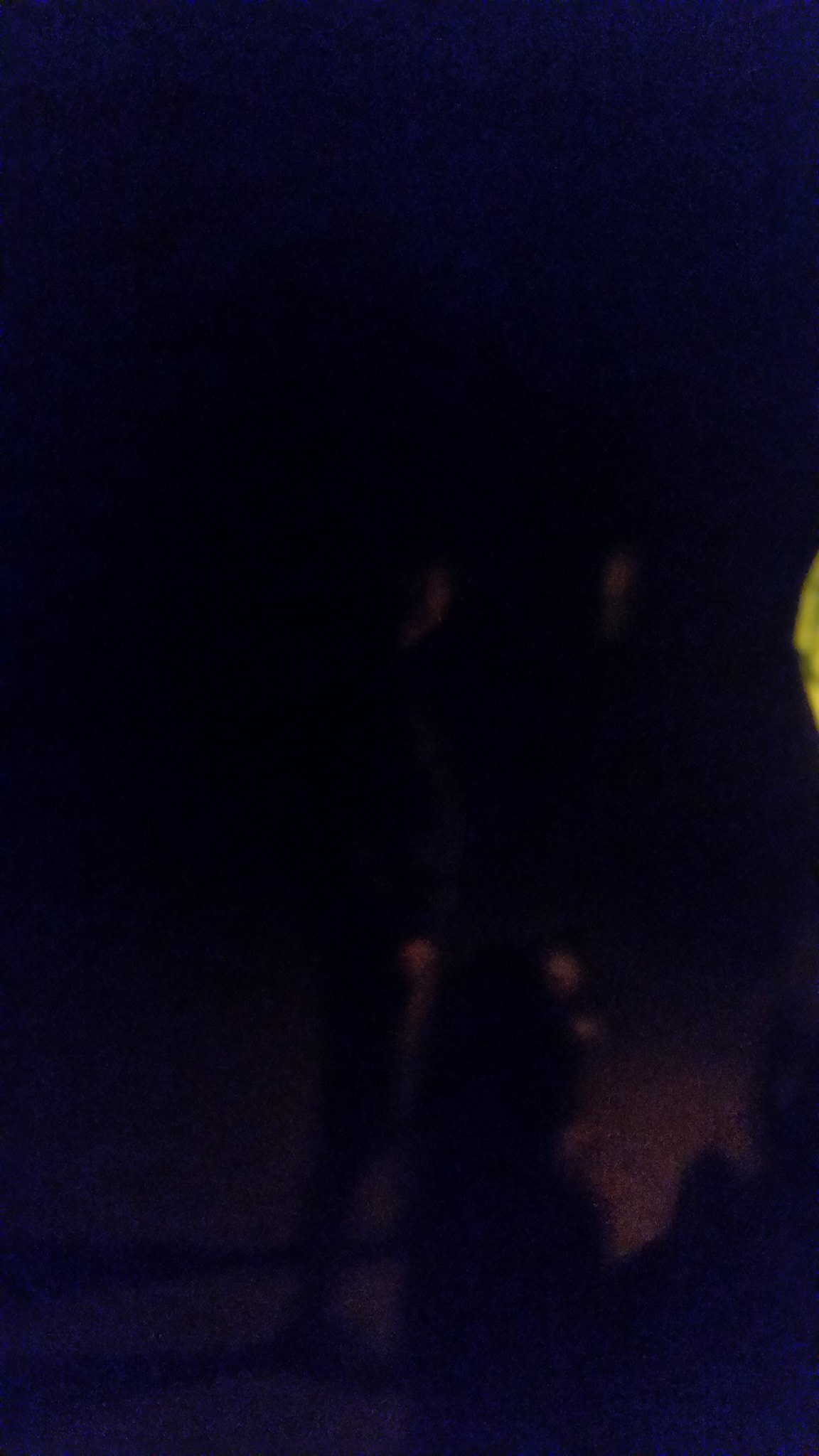The image is very poorly lit, almost entirely black, with a few elements that faintly stand out. In the center and towards the bottom right, there are four very faint orange dots. To the bottom right, there is a faint shape that vaguely resembles a pig's head facing down, with a subtle pink hue. On the right side of the image, there is a small, barely visible yellow object, and in the bottom left, there are faint shades of purple amidst the darkness.

Upon closer inspection, a person can be seen standing, their outline blurred and obscured by the poor lighting. They appear to be wearing dark-colored pants and a top, with the outline of their shoes just discernible. The person seems to be looking at something off-screen. A yellow object is almost completely cut off at the very edge of the image. Behind the person, there is a faint shadow cast on what seems to be pavement and a faint glow towards the bottom. The foreground hints at the presence of possibly two more people, but the extreme darkness makes it difficult to discern further details.